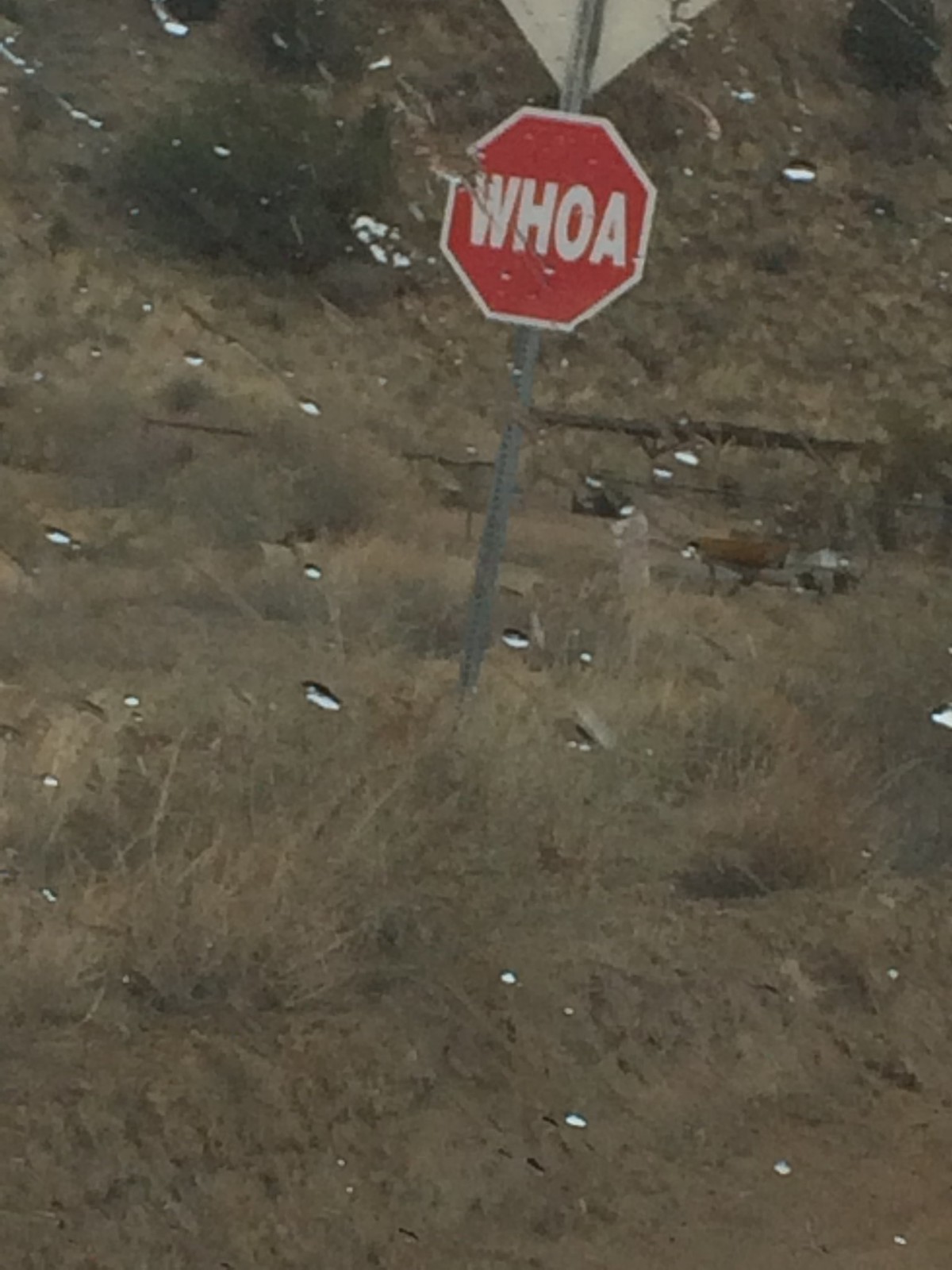The photograph appears to be taken from inside a car, capturing a roadside sign against a backdrop of parched grassland. Raindrops speckle the window, adding texture to the scene of dried, lifeless foliage stretching into the distance. The focal point of the image is a uniquely shaped hexagonal sign mounted on a post, bearing the bold red word "WOW" prominently displayed in its center.